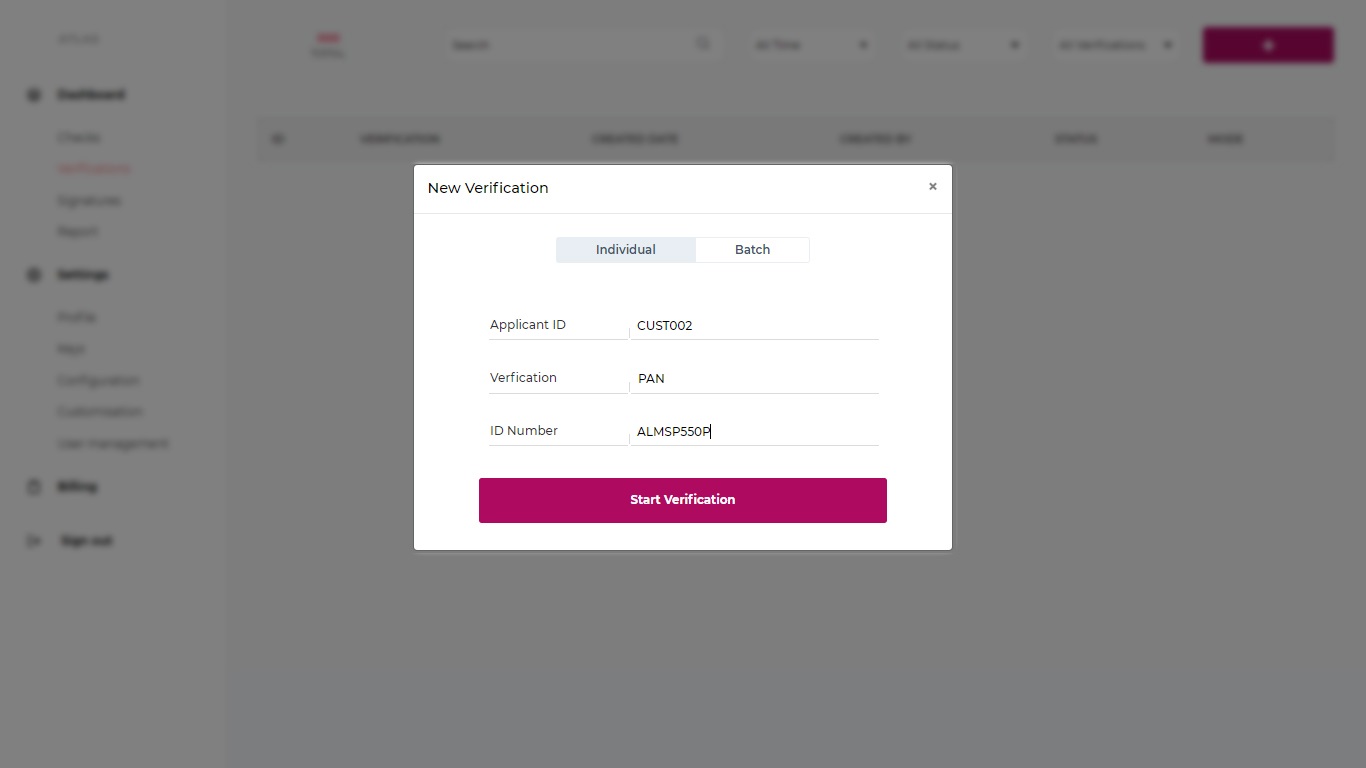The image displays a webpage with a predominantly white background. At the top of the page, there are several black navigation tabs, though their labels are unreadable due to blurriness. A notable feature is a pink button located in the top left corner, mirrored by another pink button on the top right corner.

Running down the left side of the page are multiple black text entries, which appear to be categories, with subcategories indented below them. Interspersed among these entries is one pink word, standing out against the black text. Some of the text entries are accompanied by black symbols, likely indicative of additional subcategories or options.

To the right section of the webpage, there is a large white window with several lines of black text, the contents of which are unclear.

Overlaying this page is a centered, semi-transparent pop-up box titled "New Verification," marked by a gray 'X' in its top right corner for closing the window. This pop-up includes two tabs labeled "Individual" and "Batch." Below these tabs are fields for "Applicant ID Verification" and "ID Number," which are both filled out. At the bottom of the pop-up, there's a pink "Start Verification" button with white text.